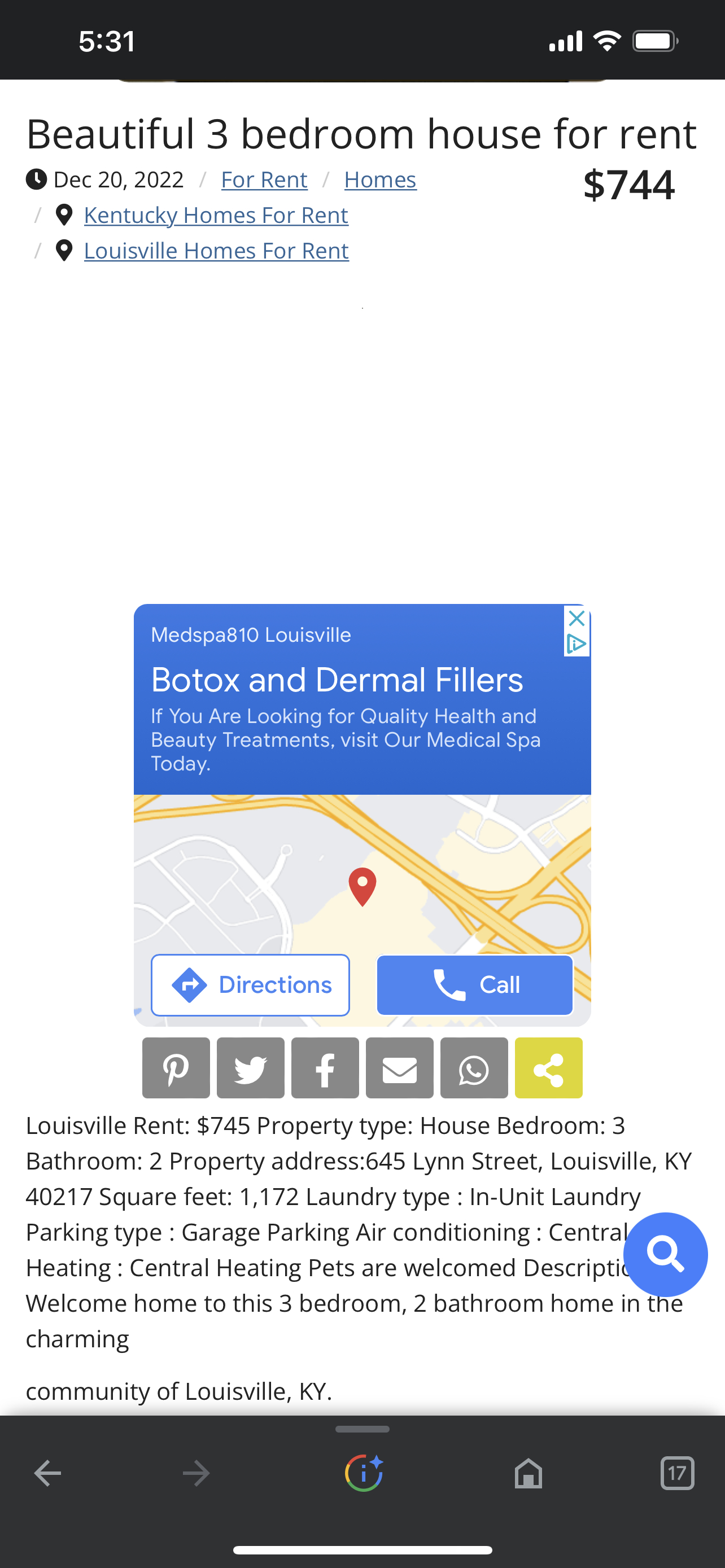This image is a screenshot taken from a smartphone, capturing a webpage displaying a real estate listing. The smartphone's status bar at the very top features a black border. On the left side, the time is shown in white font as "5:31", without specifying a.m. or p.m. On the upper right side of the status bar are icons indicating the battery level, Wi-Fi connection, and wireless network signal.

Beneath the status bar, the background of the webpage is white. The headline, written in gray font, reads "Beautiful Three-Bedroom House for Rent," with a smaller print notation of "December 20th, 2022." On the right side of the headline, the price of the house is listed as "$744."

Below the headline, in blue hyperlinks, are navigation options: "For Rent / Homes," "Kentucky Homes for Rent," and "Louisville Homes for Rent." 

Further down, there is a rectangular advertisement with a blue border at the top and white text reading "Botox and Derma Fills." This ad features an image from Google Maps.

Beneath the ad, there are social sharing buttons in gray for Pinterest, Twitter, Facebook, email, and WhatsApp.

Finally, the listing details for the property are presented. It states:
- Louisville Rent: $745
- Property Type: House
- Bedrooms: Three
- Bathrooms: Two

Additional information about the address and amenities follows this, with the background color transitioning to a very dark gray at the bottom of the screenshot.